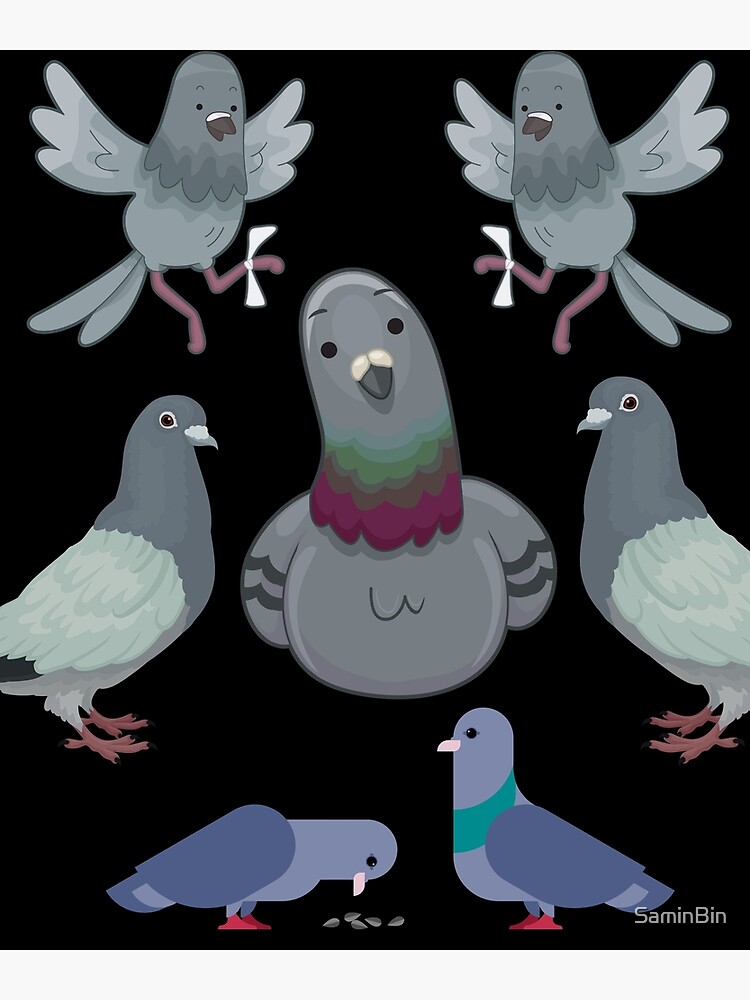The image is a vertically oriented digital illustration set against a black background, featuring seven birds. At the center, there's a prominent gray bird, possibly a mourning dove, with distinctive black stripes on its wings, white markings above its beak, and a striking purple color around its neck. Flanking this central bird on both sides are another pair of gray birds characterized by their orange feet, light gray wings, and dark gray heads, necks, and stomach areas.

At the top of the image, a pair of mirrored gray birds with pink legs can be seen, each with a white ribbon tied around one of their legs, suggesting they might be carrier pigeons. These birds have their wings spread out as if in mid-flight, possibly searching for a landing spot.

Lower in the image, on the bottom left, there is a bluish-gray bird with red feet pecking at some food on the ground, while another bluish-gray bird with a green band around its neck stands upright, facing left. Notably, the bottom right-hand corner of the image contains the text "Salmon Bin."